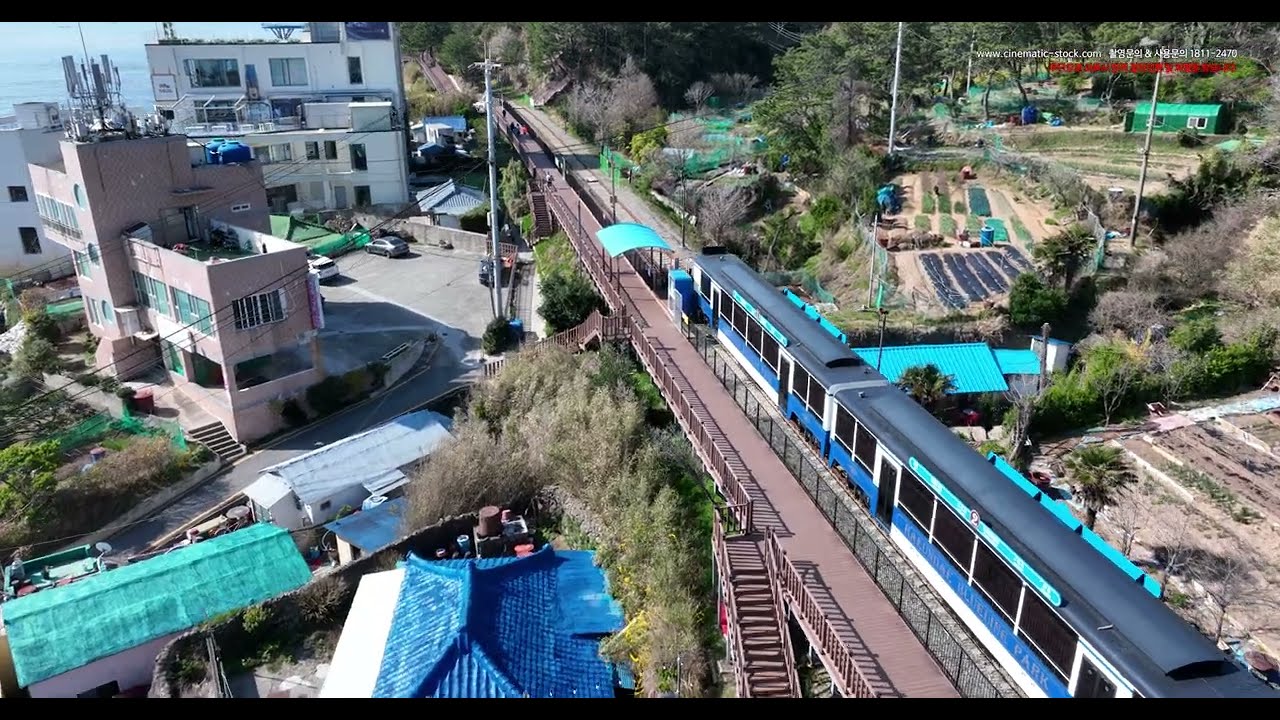This detailed aerial photograph captures a desolate train station at the center, nestled within a small, rundown village. The train, which has a black roof, blue sides with white and turquoise streaks, is stopped on brown tracks, loading passengers. The tracks run diagonally from the bottom right to the top middle of the image. A red brick pathway parallels the tracks to the left, extending upward and accessed by a staircase at the bottom.

On the left side of the image, there are several multi-story buildings, including a prominent pink building in the forefront along with two white buildings in the background, suggesting older, possibly dilapidated structures. Smaller sheds or buildings are also visible near the bottom left, close to the pedestrian walkway of the train station. Underneath or in front of a bridge to the left, more structures can be seen.

Farmland dominates the right side of the image, featuring patches of dirt and rocky terrain interspersed with rows of crops and bordered by bushes. The landscape includes several electricity poles situated near the top center. A green building is visible on a distant hill behind the train, adding to the rural, isolated atmosphere of the scene.